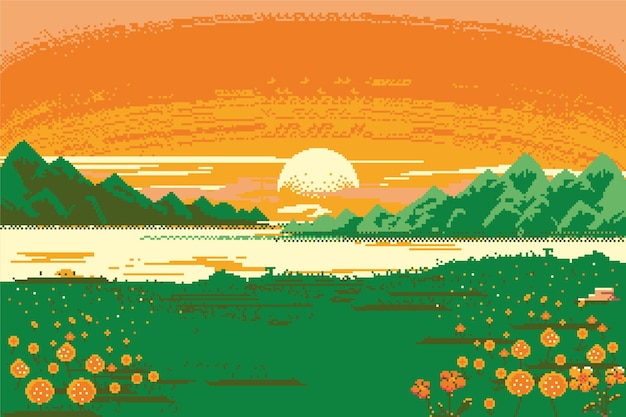This detailed, digitally created illustration evokes a nostalgic 70s vibe with its distinct color palette predominantly featuring beige, orange, and green hues. The sky, seemingly pixelated, transitions from a peachy beige at the top to a vibrant orange, decorated with textured horizontal stripes of varying shades. A white sun is seen setting into a backdrop of pinkish-beige clouds, casting bright lines across the sky. Below the sky, green mountains frame the horizon on both the left and right sides, while a yellow-tinted body of water, reflecting the sky's orange hues, stretches beneath them. In the foreground, there is a detailed representation of grass, interspersed with patches of orange flowers. These flowers vary, some adorned with white dots and others featuring yellow centers, adding a touch of vivid detail to the scene. The grassy area also contains black lines and shadows, contributing to the textured and layered feel of the illustration. The overall effect is a richly detailed, pixelated homage to vintage aesthetics.